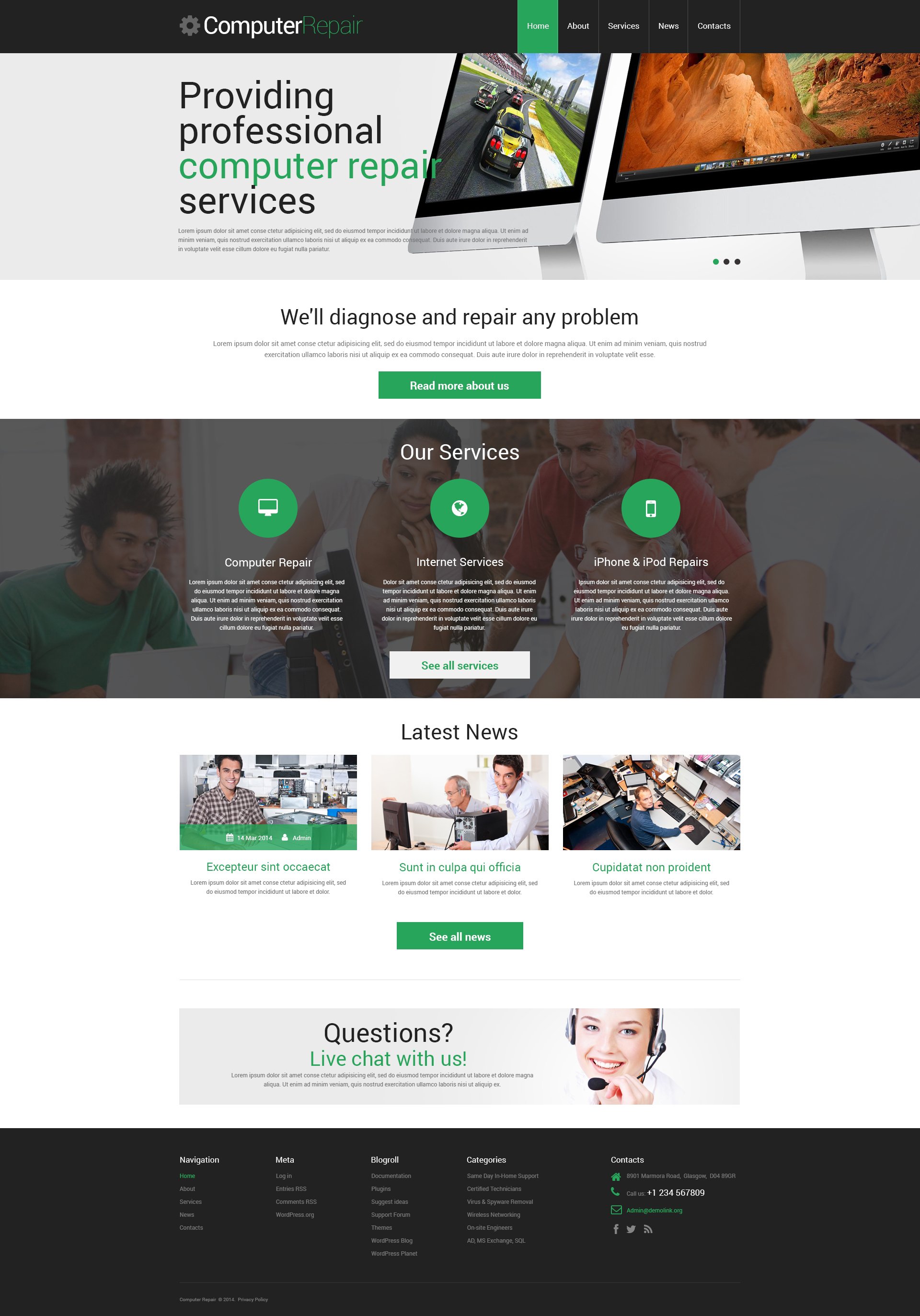Overview of a Computer Repair Website:

At the top of the website, there is a sleek black horizontal banner with the text "Computer Repair" prominently displayed in a stylish font— "computer" in white and "repair" in green. To the left of this text is a small green home icon, while to the right are icons for navigating to "About," "Services," "News," and "Contact" sections.

Directly beneath this header, a narrow horizontal banner presents the slogan "Providing Professional Computer Repair Services," with "Computer Repair" highlighted in green for emphasis. The rest of the text is in a standard black font.

The main content area features a series of images, including a computer screen displaying a racing car and another, less discernible image. Accompanying these visuals, a message promises, "We'll diagnose and repair any problem," followed by text in a foreign language, which is then concluded with a green button with a white outline inviting users to "Read More About Us."

Further down, the site introduces its services with a background showing people working at computers. This segment is also a horizontal rectangle that highlights three circular icons: "Computer Repair," "Internet Services," and "iPhone and iPod Repairs." Each icon is accompanied by brief descriptions in very small text, again in another language.

There is an option labeled "See All Services" for users wanting a comprehensive view of the offerings. Below this section is an area dedicated to the latest news, featuring images of people engaged in various activities and another "See All News" button, also in a foreign language.

A customer service feature is prominently displayed, showing a woman with a headset and promoting a "Live Chat" for any questions users might have. Lastly, the bottom of the page includes a variety of navigation links and contact telephone numbers for further assistance. This area serves as an extensive overview of the website and its functionalities.